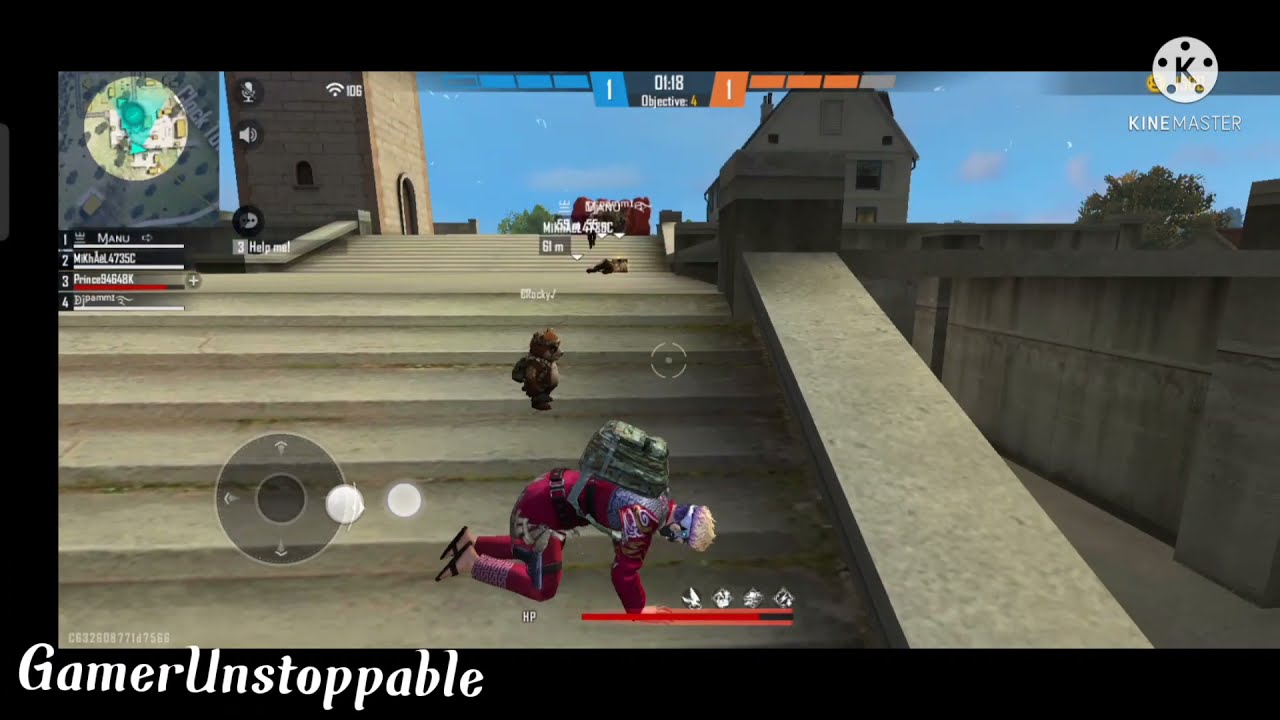The image is a screenshot from a video game titled "Gamer Unstoppable," featuring a central character clad in a wet, red jumpsuit who appears to be on his knees, possibly injured or in distress. He's equipped with a backpack that resembles a parachute or army gear. A small teddy bear stands on the stairs behind him, with more characters lined up further back. 

The setting includes a mix of architectural elements: on the right, buildings resembling mills, and on the left, a tall, brick structure, possibly part of a school or town. A stone seating area is visible along the stairs, and a large tower looms in the background. The visual design shows a blue sky, adding to the diverse backdrop.

A heads-up display (HUD) spreads across the screen, displaying various gameplay elements: a map in the upper left corner, a scoring chart with orange and blue sides at the top, gamertags, and health indicators. Text reading "Gamer Unstoppable" is positioned in the bottom left, and "Kine Master" appears in the upper right. The screenshot’s color palette includes blue, brown, gray, red, green, and black tones, suggesting a dynamic and engaging gaming atmosphere.